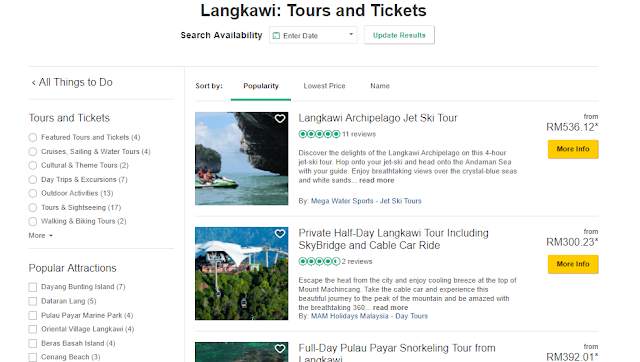Explore the stunning Langkawi Tours and Tickets options, featuring a wide variety of activities and excursions to suit every interest. Conduct a search for availability by entering your desired dates to update the results. On the left sidebar, you'll find categorized offerings such as Things to Do, Tours and Tickets, Featured Tours, Cruises and Sailing, Water Tours, Cultural and Theme Tours, Day Trips and Excursions (7), Outdoor Activities (13), Tours and Sightseeing (17), Walking and Biking Tours (2), and more categories available via a pull-down menu.

Popular attractions in the area include Da'ang Valentin Island (7 experiences), Darlene Lang (5 experiences), Putayupraya Marine Park (4 experiences), Oriental Village Langkawi (4 experiences), Bayrass Bushash Island, and Ken'ang Beach. This listing appears to be on TripAdvisor, but confirmation is needed.

A highlight is the Langkawi Archipelago Jet Ski Tour, which has received a 5-star rating from 11 reviews. This four-hour adventure allows you to discover the delights of the Langkawi Archipelago. Hop onto your jet ski and explore the Adamin Sea under the guidance of a knowledgeable tour leader.